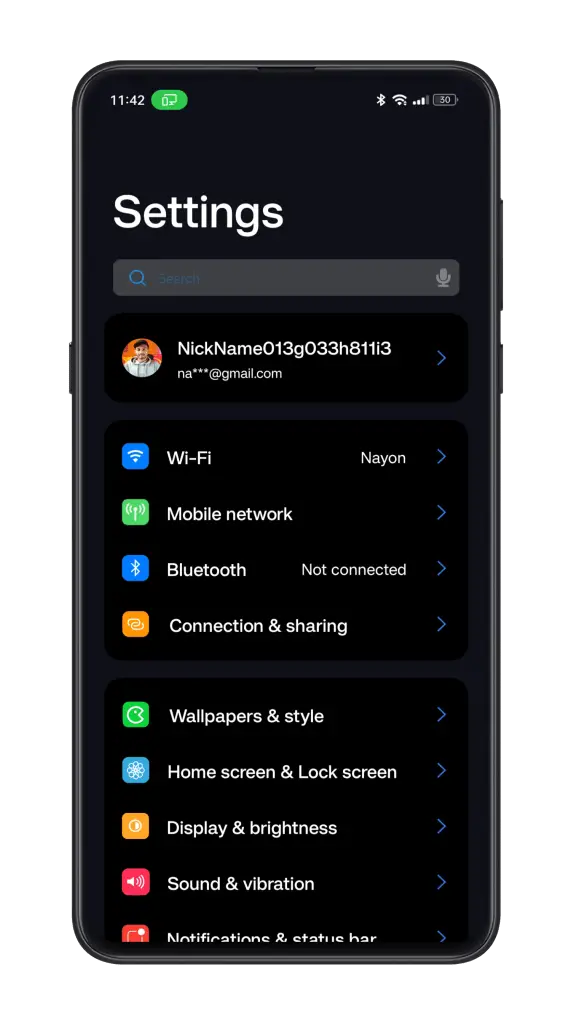Screenshot of a Mobile Phone Settings Menu

In this image, we see a screenshot taken from a mobile phone's display, featuring various elements indicative of the device's status and available options. 

At the very top-right corner of the screen, the time is shown in white text, reading "11:42." Adjacent to the time, there is a green icon depicting a computer screen. Following this, signal strength and Wi-Fi connection icons appear, along with a battery icon indicating that the battery is at 30% capacity.

Beneath these status indicators, on a black background, the word "Settings" is prominently displayed in large, capitalized white text. Directly below the title is a search bar. To the left of the search bar is a blue magnifying glass icon, and within the bar, the word "Search" is written. At the far right of the search bar, there is a gray microphone icon.

Further down, there is a circular image of a male individual wearing a gray hoodie. Next to the image, the text "nickname 013G033H811I3" is displayed, and below this, an email address partially obscured by asterisks appears, formatted as "***@gmail.com." To the right of this email address is a blue arrow, suggesting more details or options are available upon selection.

The lower portion of the screenshot includes several icons and text options for various settings:
- Wi-Fi
- Mobile Network
- Sync
- Signal
- Bluetooth
- Connection Sharing
- Wallpaper and Style
- Home Screen
- Lock Screen
- Brightness and Color
- Sound and Vibration
- Notification and Status Bar

Each of these options is accompanied by a blue arrow on the right side, indicating that tapping any of these options will allow the user to modify their respective settings.